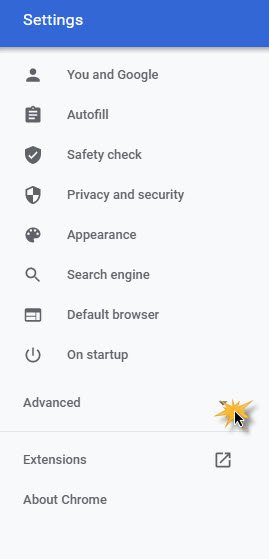This screenshot depicts a mobile phone's settings screen within an app, possibly a web browser like Chrome. The image is vertically oriented with a predominantly white background. At the top, a horizontal blue rectangular bar features the word "Settings" in white text. Below this header, various menu options are listed in a very dark gray font.

A generic user icon precedes the label "You and Google,” indicating user-specific settings. The subsequent items listed are "Autofill," "Safety Check," "Privacy and Security," "Appearance," "Search Engine," "Default Browser," and "On startup." Each option likely navigates to related sub-settings.

Further down, the word "Advanced" appears, aligned to the left and highlighted with a distinctive yellow icon resembling a sun with rays. This icon features a black arrow trimmed in white, suggesting additional options or a drop-down menu when selected. A horizontal gray line beneath "Advanced" visually separates the sections as the menu continues with "Extensions" and concludes with "About Chrome."

Overall, the image effectively organizes the settings options into a clear and structured format, with visual cues like the yellow sun icon to guide user navigation.